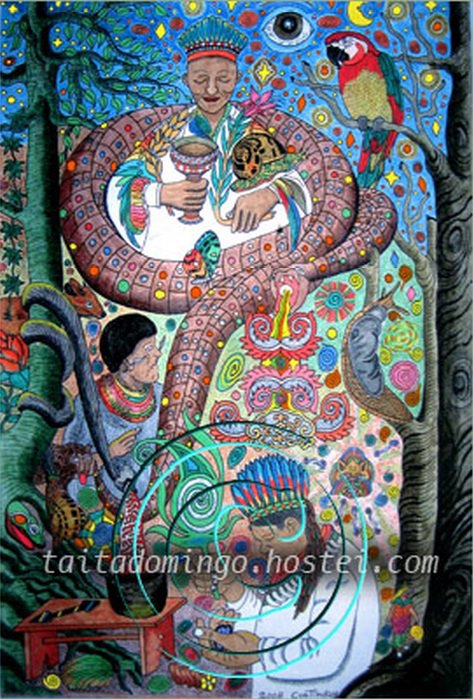The image depicts a vibrant and intricate mural that evokes the essence of a bustling Spanish marketplace with a strong South American influence. Dominated by a vivid palette of red, blue, green, and yellow, the scene is brimming with life and symbolic artwork. At the top of the mural, a blue sky frames the composition, flanked by two expressive trees - one green on the left and a darker brown and gray on the right.

Central to the mural's lively narrative are the detailed and culturally rich characters. On the left side, a man with dark skin, adorned in a white coat and a multicolored headdress of red, blue, and yellow, holds a chalice in his right hand, merging physical presence with spiritual iconography. This figure is intricately entwined with a large, jewel-encrusted serpent that meanders across the mural, adding vibrant, symbolic content.

On the right tree branch sits a parrot, adding an element of exotic wildlife to the mural. Below the central figure, another man with dark hair draped in colorful beaded necklaces over a blue shirt appears, embodying a strong South American cultural presence. The imagery continues with another person located at the bottom left, depicted with exaggerated large hands and an elaborate headdress, further enriching the narrative tapestry.

A wooden table positioned at the bottom left and numerous symbolic elements like an eye, the moon, and a snail dispersed throughout enhance the mural's abstract and whimsical nature. This intricate mural brilliantly captures the spirited and colorful essence of its cultural inspirations, culminating in a detailed and engaging piece of art. Above all, the mural bears an inscription at the bottom in white letters: 't-a-i-t-a-d-o-m-i-n-g-o dot h-o-s-t-e-r-t-e-i dot com,' anchoring the mural in a digital realm.